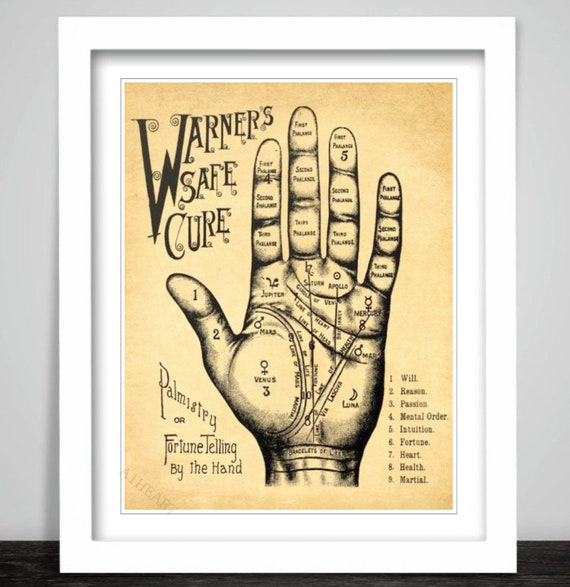This photograph showcases a framed artwork, featuring an intricate piece centered on the study of palmistry. The frame itself is a pristine white, elegantly highlighting the sepia-toned interior illustration, which is accented by detailed black ink. 

At the heart of the artwork lies an anatomically detailed image of an open hand. The wrist is positioned at the bottom, with fingers splayed upwards. The hand is meticulously annotated, with various sections and lines of the palm marked to correspond with planetary influences and astrological signs. 

Beneath the thumb, the word "Venus" is inscribed along with its associated astrological sign. Adjacent to this, the area under the pointer finger appears to be labeled with the word "Feast" or "First". On the lower right side near the wrist, "Libra" is written, accompanied by a depiction of the moon.

Continuing across the palm, beneath the ring finger are the names "Apollo" and "Saturn", while under the pinky finger, "Mercury" is clearly visible. 

The upper left corner of the artwork contains the inscription "Warner's Safe Cure", and in the lower left corner, the text reads "Palmistry or Fortune Telling by the Hand" in striking black ink. 

Overall, the image is a fascinating blend of artistic expression and the mysterious allure of palmistry, encapsulated within a classic white frame.